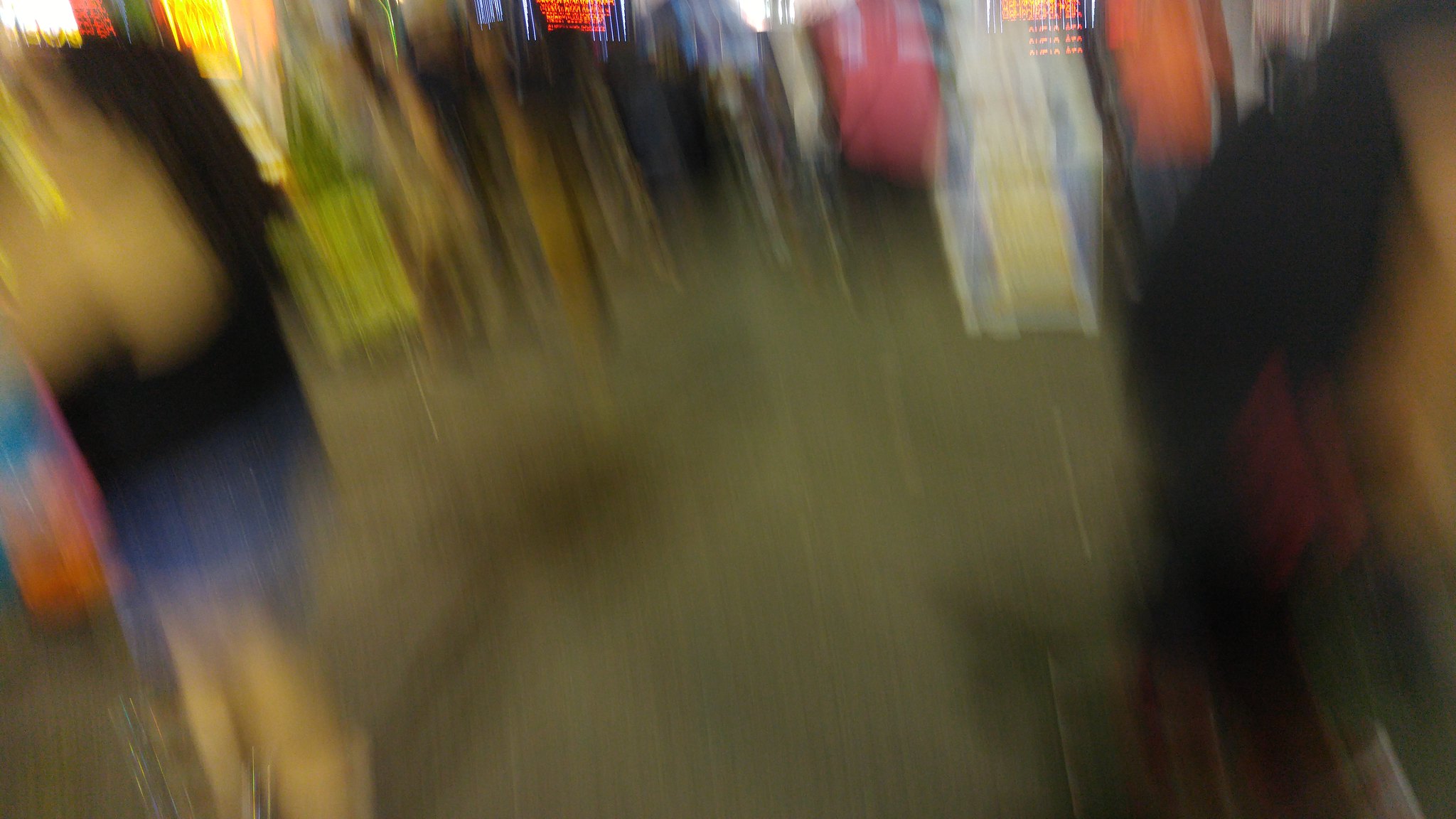This image captures a very blurry night scene that appears to be bustling with activity, possibly an outdoor arcade or carnival. Dominating the left side, there's a blurry figure that might be a person wearing a black, sleeveless top and blue skirt or jean shorts, with something yellow and a red purse visible against their side. This individual seems to have long brown hair. To the right of this person, several indistinct figures can be identified, contributing to the chaotic, lively atmosphere. The background is vibrant with a multitude of colorful lights—orange, yellow, green, pink, and blue—possibly neon signs or lighting from various stalls, games, or shopping districts. The ground underfoot looks to be a simple brown surface. Far in the distance, there's a screen emitting red lighting, adding to the festive yet blurred scenery. The overall composition suggests a night-time street scene filled with people and colorful lights, immersed in motion blur.